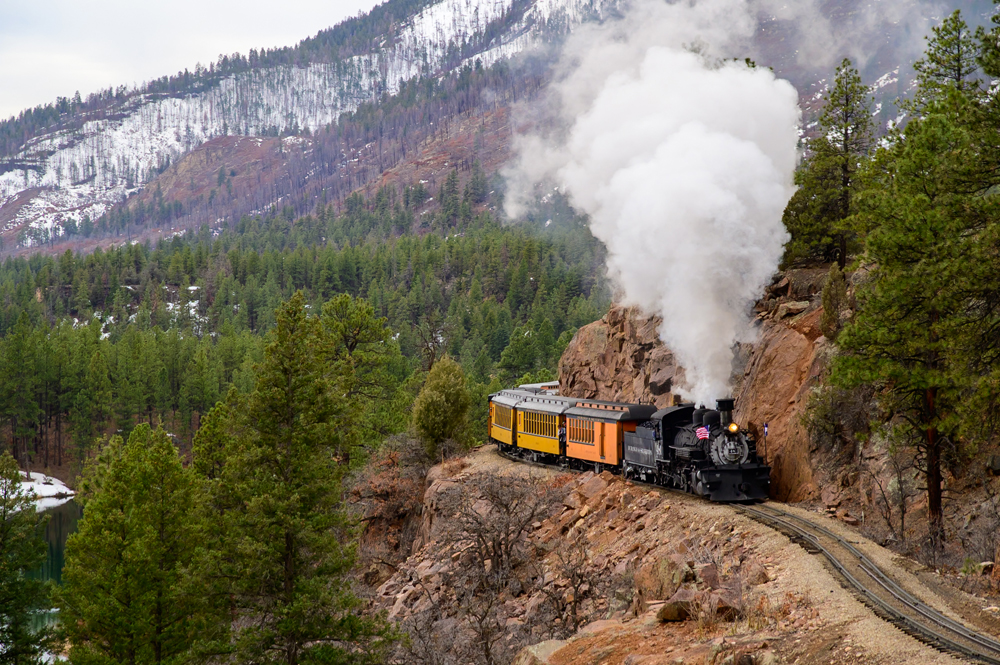In this detailed image, a steam engine train is navigating a winding railway that skirts the edge of a rugged cliff, descending towards the bottom right of the frame. The train's engine, predominantly black with some pink accents and a bright yellow headlight, emits a large puff of steam. Behind the engine, there are four cars: the first is a vivid orange, followed by two lighter orange to yellow cars, and finally, a caboose.

The rocky cliffside is visible, lined with trees—some bare and others lush with leaves or fir needles—that stretch into the distant background. The landscape transitions into a substantial snow-dusted mountain on the left, sparsely covered with snow, suggesting a mild winter scene. The mountain's base and its slopes exhibit a variety of tree species, with some showcasing red and orange hues. Towards the right of the train, a dense forest of tall, elegant evergreen trees stands.

Above, the sky is partly visible, filled with clouds, adding to the dramatic scene of the train journeying through this picturesque, yet formidable, natural landscape.